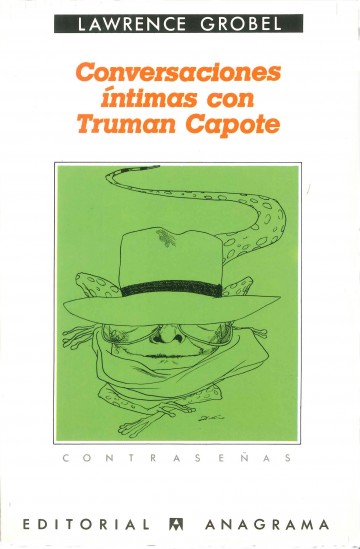The cover image of a Spanish-language edition of "Intimate Conversations with Truman Capote" by Lawrence Grobel features a distinctive illustration. It consists of a green rectangular background, slightly darker than lime or olive green, with a black ink drawing. Dominating the image is a surreal figure that blends a human and a reptile. The figure wears a hat similar to one paired with a trench coat, characterized by a square top and a wide, 360-degree brim with a black sash, obscuring its eyes. The figure’s head, which bears a wide face, sprouts two diagonally positioned cat-like ears that resemble pickles. The body transforms into a creature with frog legs and a tail, which is dotted in an angular pattern. The cover is titled "Conversaciones Íntimas con Truman Capote" in orange, serif, italicized font. Above the image, in a black rectangle, "Lawrence Grobel" is inscribed in white, all-caps, sans-serif font. Below the illustration, the text reads "Contraseñas," followed by "Editorial Anagrama" in black letters and the publisher's insignia, also in all-caps, sans-serif font. There is an artist's signature beneath the illustration, though it is too small to decipher.